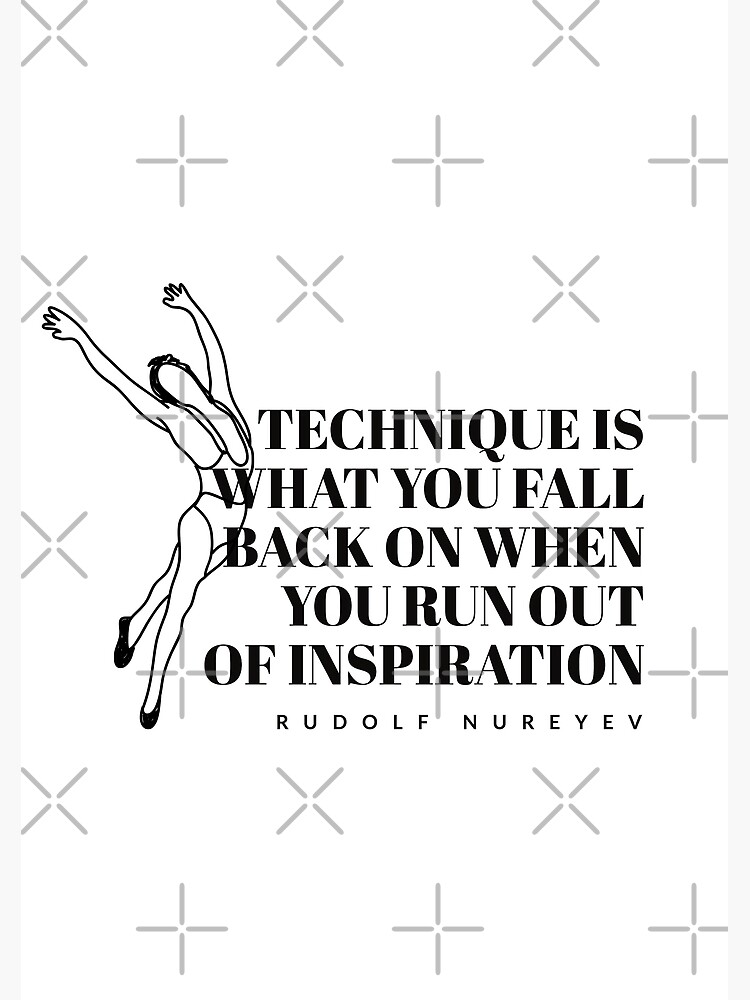The image features a white background with an alternating pattern of gray X's and plus signs, arranged in horizontal lines across the entire picture. In the center, there is a cartoon-like illustration of an individual performing a dance move, which appears to be ballet or possibly a gymnastic routine. This person, who lacks facial features, is depicted with short black hair and is dressed in a leotard with thin straps, resembling a bathing suit, and wearing what look like black ballet shoes. They are posed with one leg extended behind the other, their arms raised above their head, and their back arched, suggesting a graceful movement. The person has four digits on each hand. To the right of the figure, in black text, is the quote: "Technique is what you fall back on when you run out of inspiration. Rudolf Nureyev."